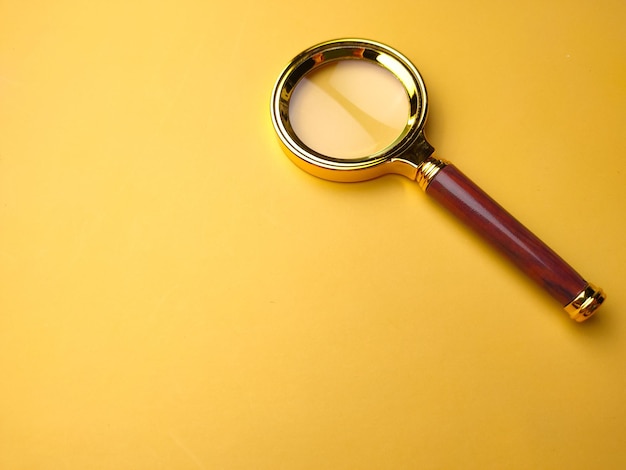This is a detailed image of a magnifying glass lying on a bright yellow background. The glass lens reflects the yellow surface, indicating its transparency. The magnifying glass's head is encased in gold metal trim, giving it a luxurious appearance. The handle extends diagonally to the right edge of the image and is dark brown with subtle, almost wood-like swirls, suggesting a two-tone pattern. The handle features gold accents at both the joint and the tip, enhancing its elegant design. This simple, yet striking photograph highlights the magnifying glass against the solid yellow backdrop with no other objects present, emphasizing its form and craftsmanship.